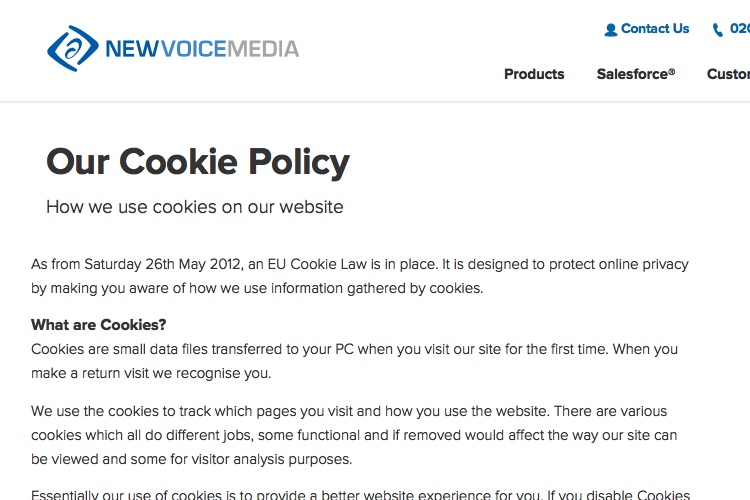Screenshot from a website displaying a cookie policy:

The image showcases a website screenshot set against a white background with primarily black text. In the upper left-hand corner, there is a logo resembling a diamond shape with a blue swirl in the middle. This logo is accompanied by the text "new voice" in blue and "media" in grey, formatted as a single word, "newvoicemedia."

In the upper right-hand corner, the options "Contact Us" colored in blue, along with icons representing a telephone and a head-and-shoulders silhouette of a person, are visible. Next to these icons, the partial text "021" is present, suggesting that the full phone number is cut off.

Below this header section is a thin horizontal grey line. Underneath, aligned to the left, there is a large heading in black text: "Our Cookie Policy" followed by subheadings and explanatory text. The heading is followed by the introduction, "How we use cookies on our website."

The content begins with a date, "As from Saturday, 25th May 2012," and mentions the implementation of the EU cookie law aimed at protecting online privacy by informing users about how cookie-related information is utilized.

A bold subheading, "What are cookies?" precedes the explanation: "Cookies are small data files transferred to your PC when you visit our site for the first time. When you make a return visit, we recognise you. We use the cookies to track which pages you visit and how you use the website." 

Additional text outlines the varying functions of different cookies, specifying that some are essential for the site's functionality and visitor analysis. The text that can still be read mentions, "Essentially, our use of cookies is to provide a better website experience for you if you disable cookies," before being cut off.

The overall visual experience indicates that some parts of the right side, including additional text, are not fully visible, suggesting the screenshot captures only a portion of the entire webpage.